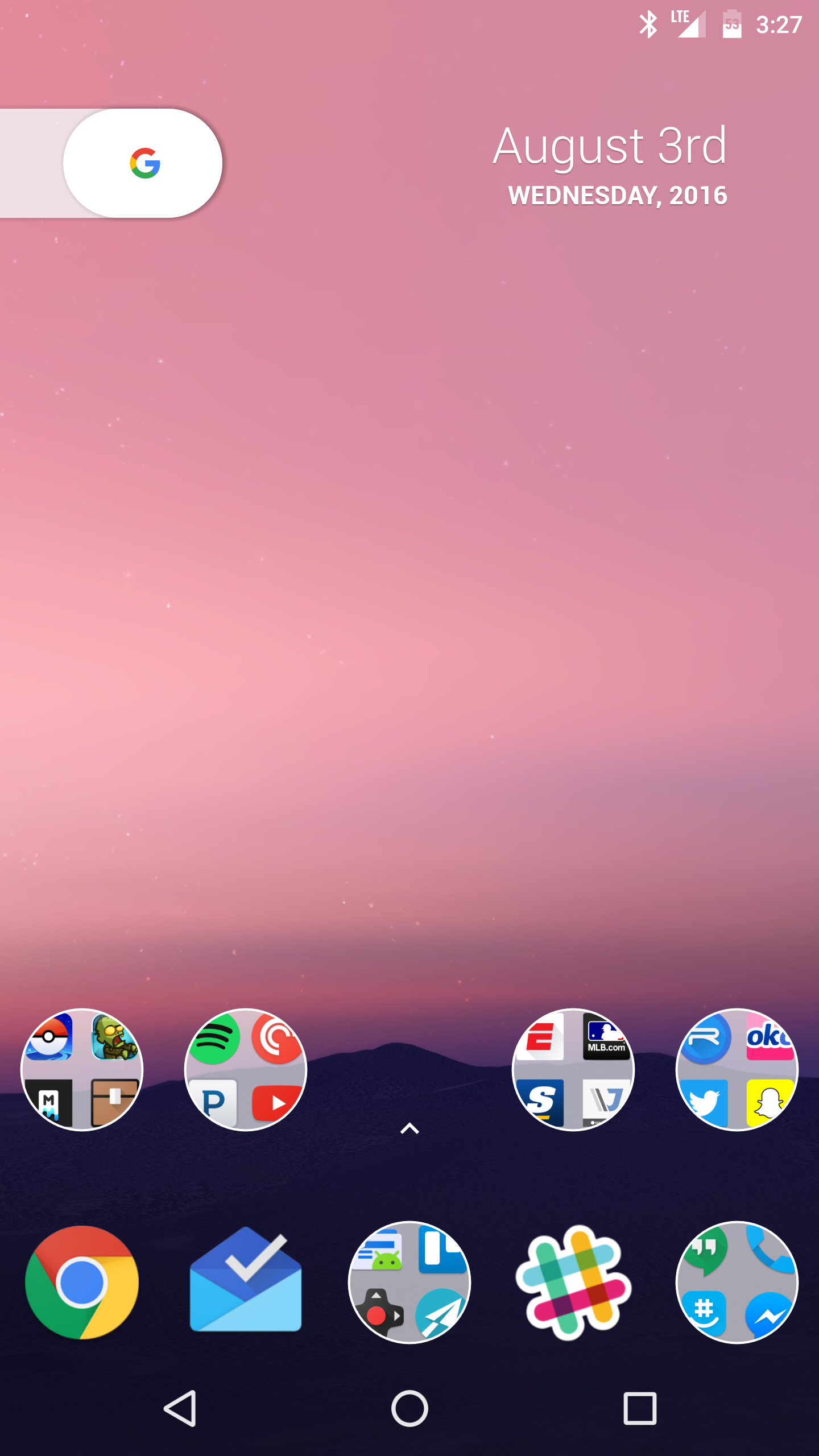The image is a screenshot from the home screen of a smartphone, showcasing a beautifully detailed background set against the top three-quarters of the screen. The background depicts a serene sky, potentially during a sunrise or sunset, characterized by solid shades of pink at the top. Below, the sky transitions into clouds with delicate gradations of blue and very light shades of lavender.

In the top-right corner of the screen, the time is displayed as 3:37 PM, accompanied by various status icons: a half-charged battery icon, an LTE icon indicating wireless connection, a Bluetooth icon, and the date shown as "August 3RD, Wednesday 2016," marking this screenshot as being from several years ago.

On the left side of the upper section, opposite the date, there is a white oval encasing the letter "G" in Google's signature colors: red, yellow, green, and blue.

The bottom portion of the home screen features a darkened area resembling mountains beneath the radiant sky. Two rows of app folders are neatly arranged, each folder represented by small circular icons. Among these, recognizable app icons such as Snapchat (yellow), Twitter (blue from that era), Spotify (green), and YouTube (red) can be identified.

At the very bottom of the screen, prominent app icons include Google Chrome on the left, an email app, and three additional app folders, completing the well-organized digital landscape of this home screen.